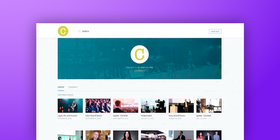This image is a partially loaded screenshot displaying the top segment of a web page. The background of the page is visually striking, featuring a gradient that transitions from bright purple on the left to a softer blue on the right. 

In the foreground, there is a large white rectangle that is not fully visible, making the text within it difficult to discern. At the top left corner of this rectangle, there is a small, circular emblem shaded in a yellowish-green hue. This circle might contain the letter "C" in white, although its small size makes it hard to confirm.

Beneath this emblem is a wide, rectangular banner with an aquatic, tealish-blue color. This banner also features a white circle in its center, prominently displaying the letter "C". Below this banner, there is a narrow strip of white space, leading to two rows of images. 

The first row consists of seven individual pictures, each exhibiting a variety of vibrant colors, suggesting they may be colorful photographs or graphics. A second, partially visible row of similar images appears just below, though the bottom portion of these images is cut off due to the incomplete loading of the page. The overall effect is one of a bright and visually engaging layout, designed to capture the observer's attention.